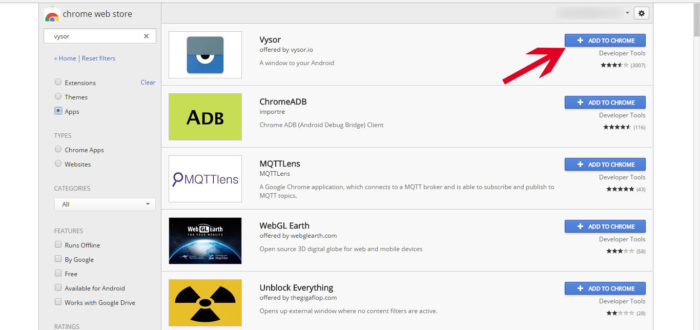The image displays the Chrome Web Store interface. In the upper left corner, the text "Chrome Web Store" is written in lowercase, dark gray font. Adjacent to it is the Google Chrome Web Store logo. Beneath this header is a prominent search box, within which the term "BYSOR" has been entered, indicating an ongoing search for this keyword. Below the search box are several navigational buttons, including options for "Home" and "Reset filters." Users can further specify their search criteria by selecting from categories such as themes or apps, and filter by type, like websites or Chrome apps.

A dropdown menu is available for more granular category selection, accompanied by various feature filters towards the bottom of the search panel, allowing users to refine results based on attributes like compatibility with Android, whether the content is free, if it is Google-authored, or its offline capabilities.

The primary search result displayed is for "BYSOR," provided by bysor.io, described as "a window to your Android." To the right of this result, a prominent blue button labeled "Add to Chrome" is highlighted by a large red arrow, indicating the action required to add the extension to the browser. Additionally, four other search results are shown, which appear unrelated to the keyword "BYSOR."